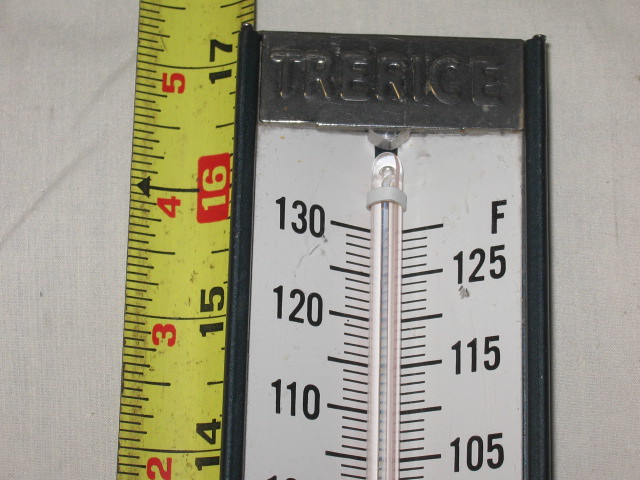This detailed photograph showcases the top portion of a mercury thermometer used for gauging ambient temperatures, either outdoor or indoor, rather than body temperature. Positioned against a pristine white background, the thermometer features a sleek black base and a metallic top, likely crafted from stainless steel, that is inscribed with the brand name “TRERICIE.” The visible temperature scale on the thermometer starts at 105 degrees Fahrenheit and extends to 130 degrees, with the markings arranged as follows: on the right side, the increments are 105, 115, 125, and 130, each accompanied by an “F” for Fahrenheit, while on the left side, the increments are 110, 120, and 130. Adjacent to the thermometer, a yellow metal measuring tape runs parallel, beginning just below the 2-inch mark and extending slightly beyond the 5-inch mark. The measuring tape distinctly displays the numerals 2, 3, 4, and 5, meticulously detailing the length of the thermometer segment visible in the photograph.